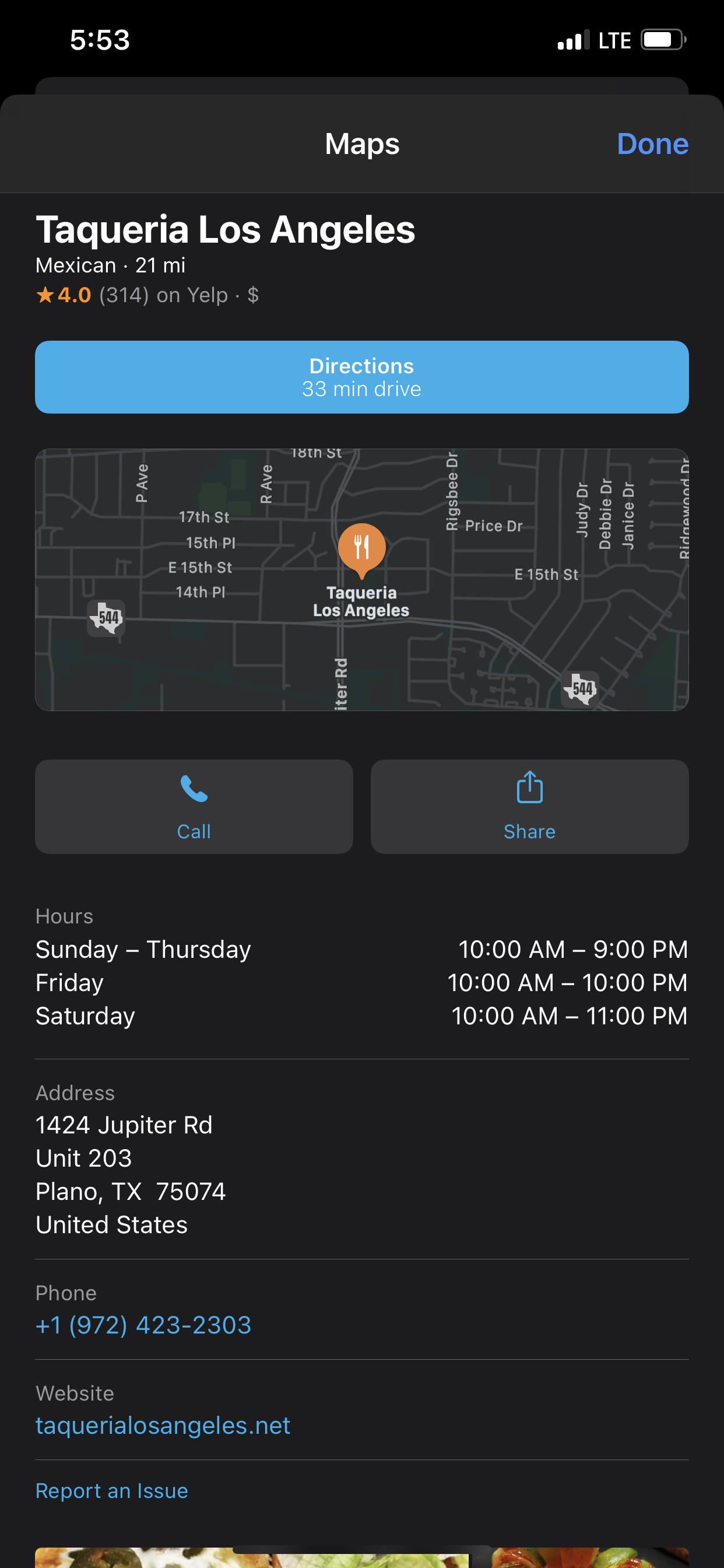The screenshot displays a smartphone running a map application, specifically showing directions to a restaurant named Tequila, Los Angeles. At the top of the screen, the application header reads "Maps". Beneath this, the search query for "Tequila, Los Angeles" is visible. The displayed address for the restaurant is 1424 Jupiter Road, Unit 203, Plano, Texas, 75074, United States, and its website is tequilalosangeles.net. 

Midway through the screenshot, the operational hours for the restaurant are detailed: Sunday through Thursday, 10 a.m. to 9 p.m.; Friday, 10 a.m. to 10 p.m.; and Saturday, 10 a.m. to 11 p.m. The top portion of the map provides a visual representation of the route, alongside a button that, when pressed, offers detailed driving directions. According to the map, it would take approximately 33 minutes to drive to this location from the current position of the user.